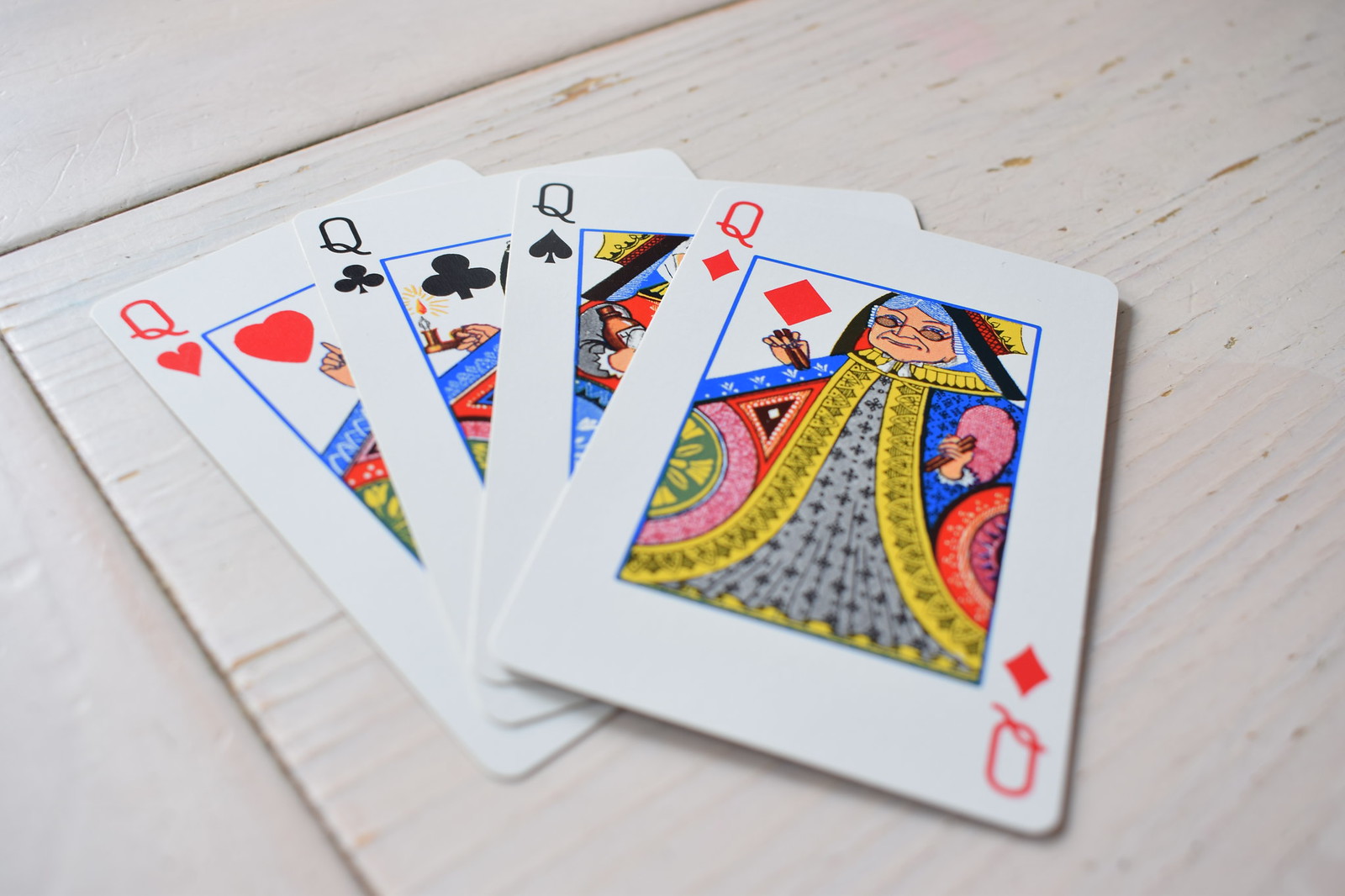This detailed photograph features a fanned arrangement of four playing cards, each representing one of the queens from a standard deck. The cards lie flat on a rustic, white-painted wooden surface that shows signs of wear, revealing the natural wood grain in some areas. The featured queens include the Queen of Diamonds, Queen of Spades, Queen of Clubs, and Queen of Hearts, arranged with the Queen of Diamonds on top. Each queen card is intricately designed, with the Queen of Diamonds showcasing a woman dressed in an elaborate, multi-colored Middle Ages gown adorned with gold, pink, red, green, and blue accents. The card suits are distinct in their traditional colors: the diamond and heart in red, and the spade and club in black. The backdrop includes a similarly painted white wall, enhancing the vintage and rustic aesthetic of the composition.